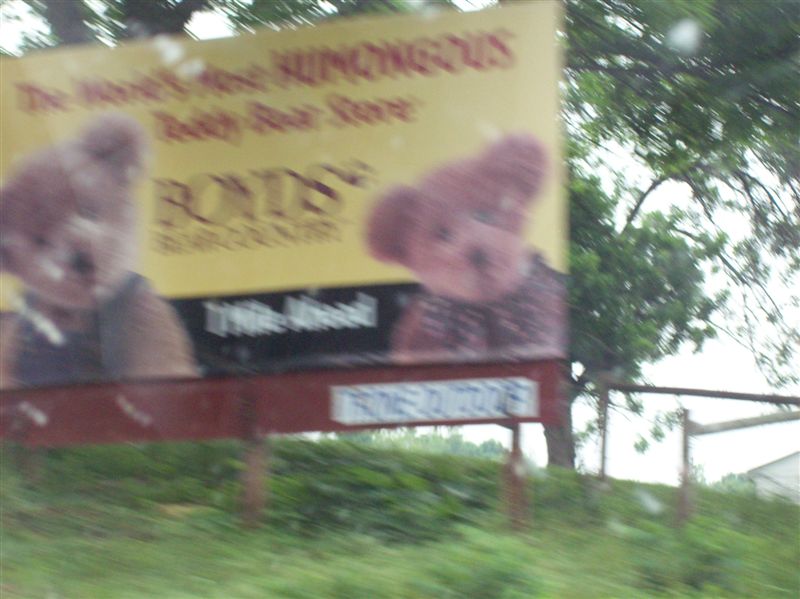This image captures a hillside billboard, distinct from the tall sky-high signs, securely set into the ground with slight elevation. The photo appears to be taken in motion, likely from a moving vehicle, resulting in a noticeable blur and partial cropping of the billboard. The sign features two classic cotton brown teddy bears, one dressed in overalls and the other wearing an indistinguishable outfit. The billboard advertises "The World's First Humongous Teddy Bear Store" followed by the name "Bonds" in red text. The slant of the hill and the overall composition suggest a dynamic and candid snapshot.